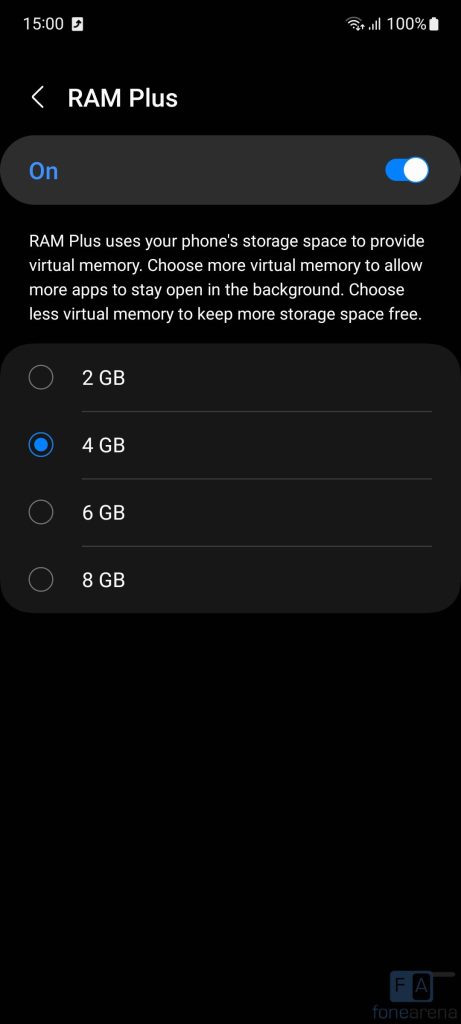The image displays a configuration interface for "RAM Plus" at the top left corner, indicated by an arrow pointing left. Below the header, there's a box with blue text that shows the feature is turned on through a slider bar. The text within the box explains that "RAM Plus" utilizes phone storage space to create virtual memory, allowing more applications to remain open in the background by choosing higher virtual memory or conserving storage space by selecting lower virtual memory.

Below the explanatory text is a selection list for adjusting the amount of RAM, with options listed as 2GB, 4GB, 6GB, and 8GB. Each option is accompanied by a selectable circle, and the 4GB option is highlighted, indicated by a filled blue circle. In the bottom right corner, there's a blue translate symbol. Other notable elements include "15" in the top left corner and a battery indicator showing 100% in the top right corner. The overall layout is clean, with no additional elements apparent in the image.